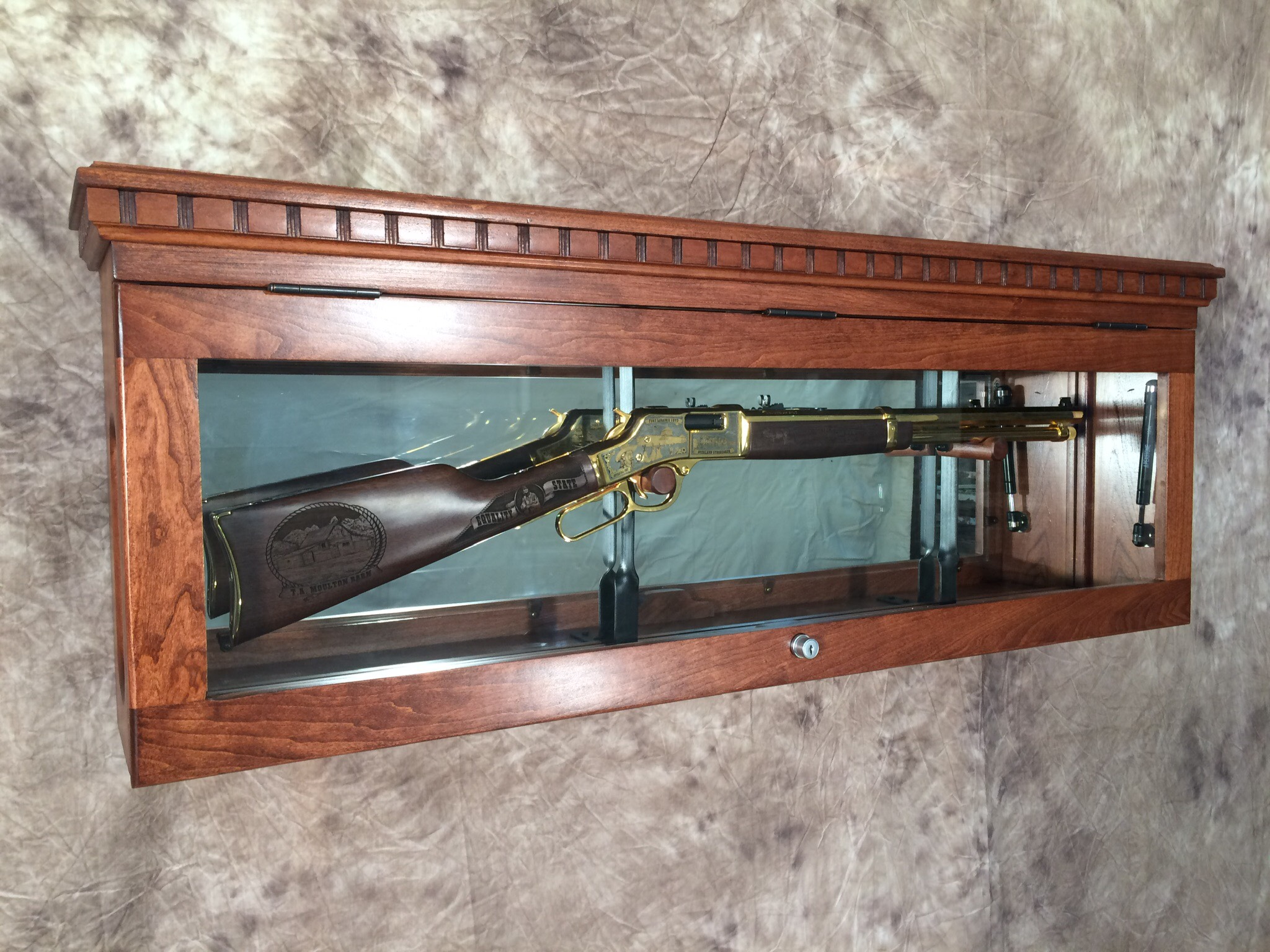The image displays an intricately designed wooden gun case mounted within a gray marbled wall, suggestive of an indoor setting, possibly a museum. The case features a glass front with three hinges at the top and a locking mechanism at the bottom center on the wooden part. Within the case is an antique rifle, mounted securely with several fixtures to prevent movement. The rifle, characterized by its dark, metallic, and rubbed appearance, boasts gold accents, with the firing mechanism and parts of the barrel adorned in gold. The stock of the rifle is dark wood, featuring a detailed design including an image that appears to depict a house with trees behind it, though the accompanying text is too small to discern. The case also has a fancy top and hydraulic hinges for smooth opening and closing.